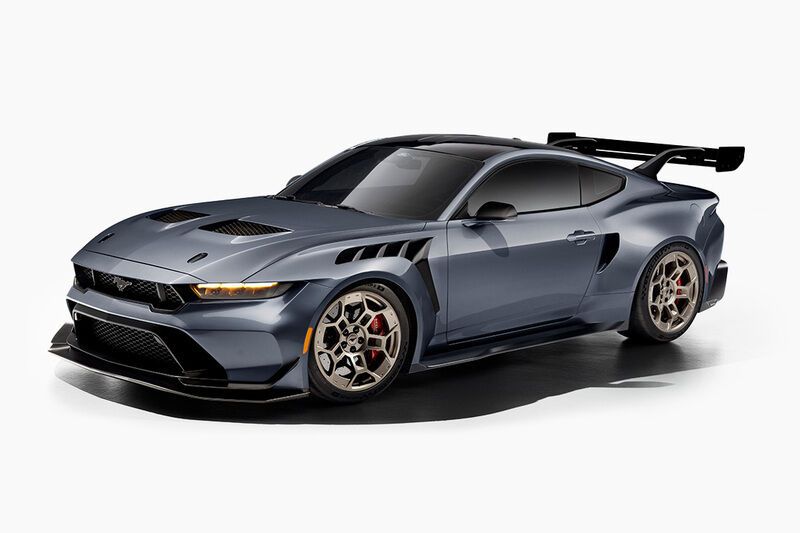The image showcases a dark blue Mustang sports car against a stark white background, positioned horizontally with the front facing the left. The Mustang, possibly a modern model, boasts an array of intricate details starting with prominently visible Mustang logos and a distinctive grille giving it an aggressive, snarl-like front profile. The car features tinted windows and sleek black accents, emphasizing its modern aesthetics.

Air vents are strategically placed across the vehicle, including above the front wheels, on the hood, and at the front of the rear fender—enhancing its aerodynamics and hinting at a powerful engine under the hood. The wheels are adorned with elaborate rims, adding to its sophisticated appearance. Notably, the rear end sports a substantial spoiler suspended above the trunk, further contributing to its sporty look.